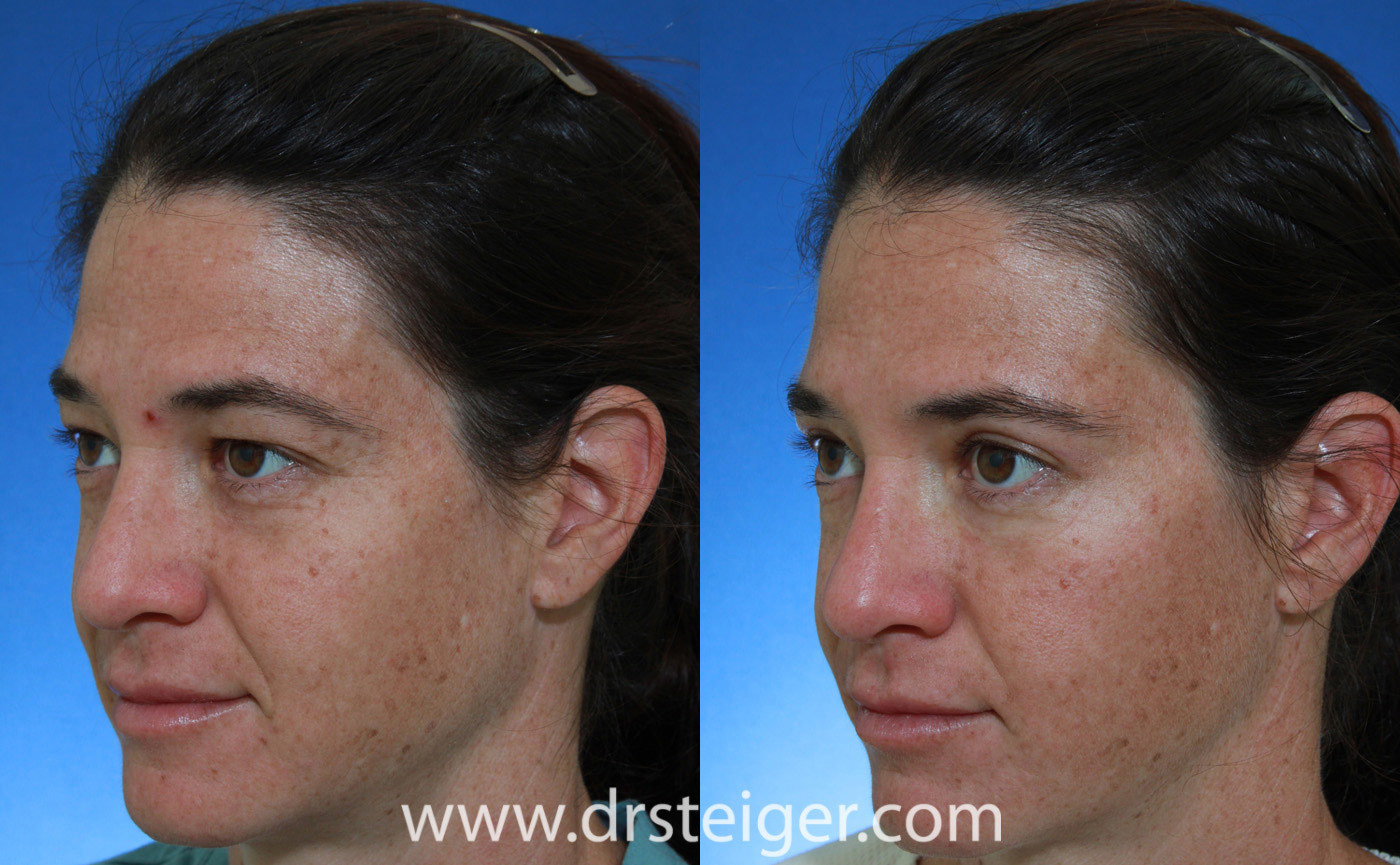The image showcases a before and after comparison of the same woman, likely depicting the results of a treatment. Both sides feature a woman with long, black hair adorned with a silver barrette. Her face has a light complexion and she has brown eyes, freckles, and a slightly smiling, closed mouth in both images. In the left image, the woman’s eyes are not as widely opened as in the right image, and she has visible red blemishes, including a red sore near her eyebrow and other pimples and pigmentation. In the right image, her skin appears smoother with reduced redness and fewer blemishes. The background of the image has a blue gradient that lightens towards the bottom. A watermark at the bottom center reads "www.drsteiger.com," suggesting a possible connection to a cosmetic or skin treatment by Dr. Steiger.